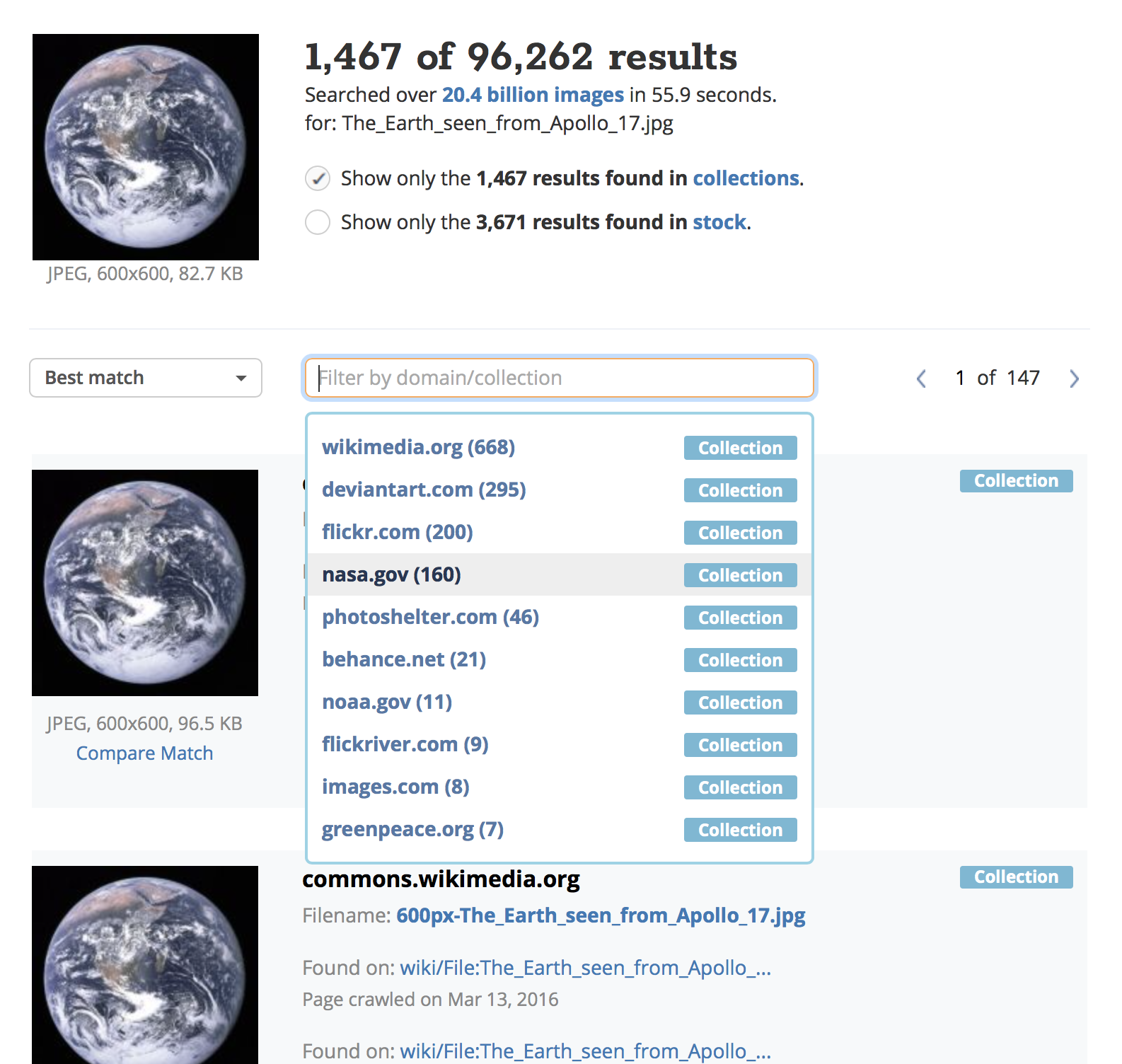The image depicts a search result page, specifically tailored for finding images of Earth, seen from the Apollo 17 mission. The layout is as follows:

- **Left Section**: A prominent image of the Earth set against a black background. The image is labeled as "JPEG" and its dimensions are 600 by 682.7 kilobytes.
- **Right Section**: Displays detailed search metrics:
  - Shows that there are 1,467 of 96,262 results available, which were searched over a database of 20.4 billion images in 55.9 seconds for the term "the_earth_seen_from_Apollo_17.JPG."
  - There's a checkbox for "show only the 1,467 results in collections," which is checked.
  - Another checkbox for "show only the 367 and one results found in stock," which is unchecked.
  
Below this:
- A dropdown menu labeled "Best Match," which displays another image similar to the one on the left, albeit labeled "JPEG 600 by 600 bits, 96.5 kilobits, Compare Match."
- A filter option labeled "Filter by domain/collection," highlighting several domains with "nasa.gov" being selected. The selected domain is marked in black with a gray background, whereas the other options are displayed as blue links.
  
On the side, there is a button labeled "Collection" in white text, set against a turquoise background. 

The page is predominantly white with specific highlighted sections in black or gray, and an interactive button on the right-hand side.